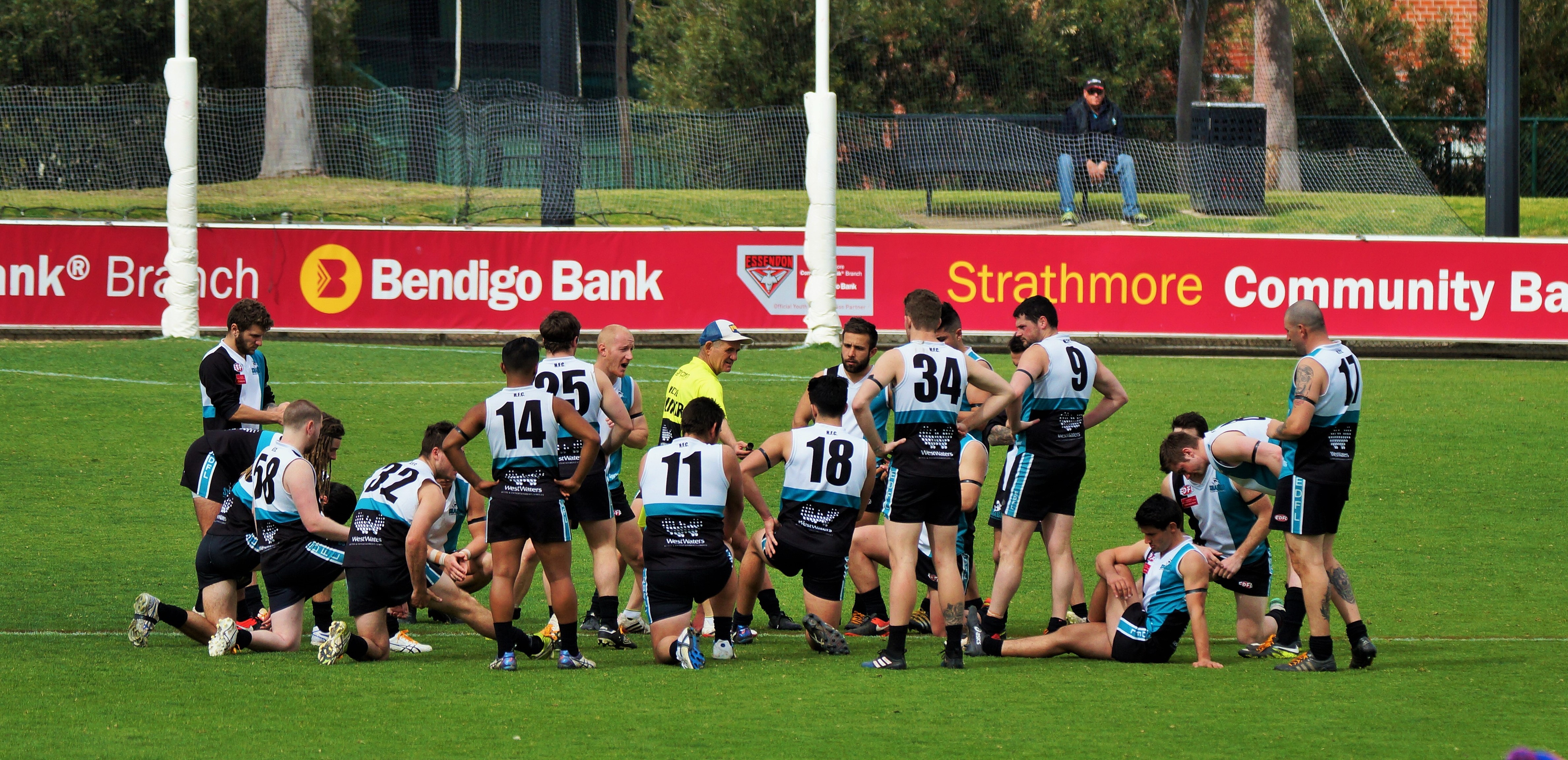The image captures a soccer team comprising around 15 male athletes, some standing, kneeling, or sitting on a green turf field. The players are wearing black shorts and white tops with black numbering, ranging from numbers like 11, 14, 17, and 32. Central to the scene is a coach, distinguished by his yellow shirt and blue and white ball cap, who is addressing the group; an assistant coach stands nearby. The background features a prominent red banner running along a perimeter fence, displaying "Strathmore Community Bank" and "Bendigo Bank." A wire fence is just visible above this banner. Additionally, there is a man seated on a bench further back, attentively observing the team.